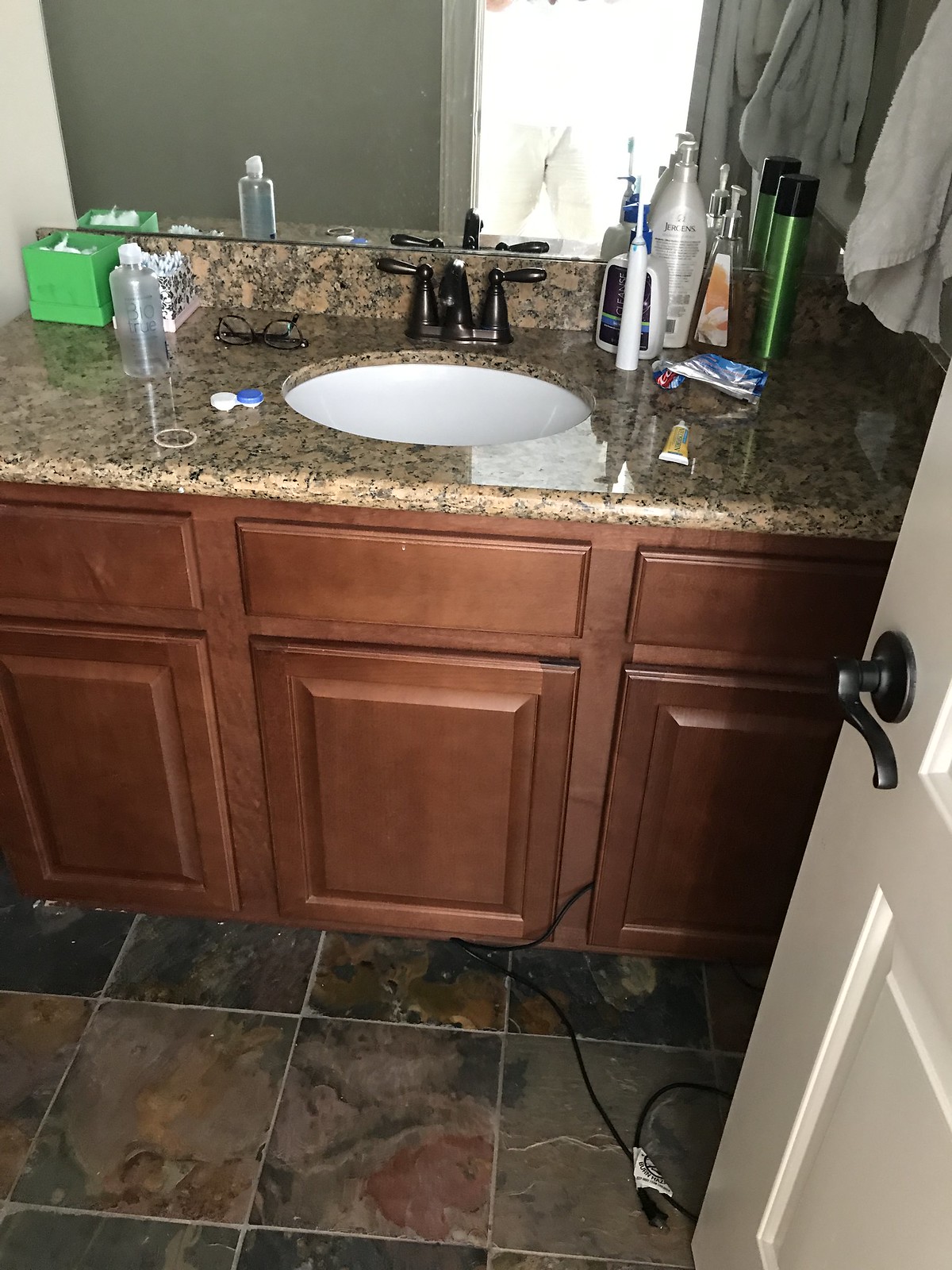This image captures the interior of a well-appointed bathroom, seen through an open door with a black handle. The door itself is white. Stepping inside, the left wall is painted a sophisticated gray, offering a modern touch to the space. Dominating this wall is a rectangular, white-framed mirror, placed directly above a sleek, round-edged rectangular sink. 

The sink is integrated into a luxurious brown granite countertop, which rests on elegant brown cabinets. On this countertop, various personal care items are neatly arranged: bottles of lotion, an electric toothbrush, and a spray bottle that features a striking black and green color scheme. Also present is a green container situated further back on the counter. A pristine white towel hangs conveniently close to the sink, adding to the bathroom's clean look.

One of the cabinet doors is slightly ajar, revealing the corner of a carton inside. The entire setup speaks to a blend of practicality and style, highlighting the bathroom's well-thought-out design elements.